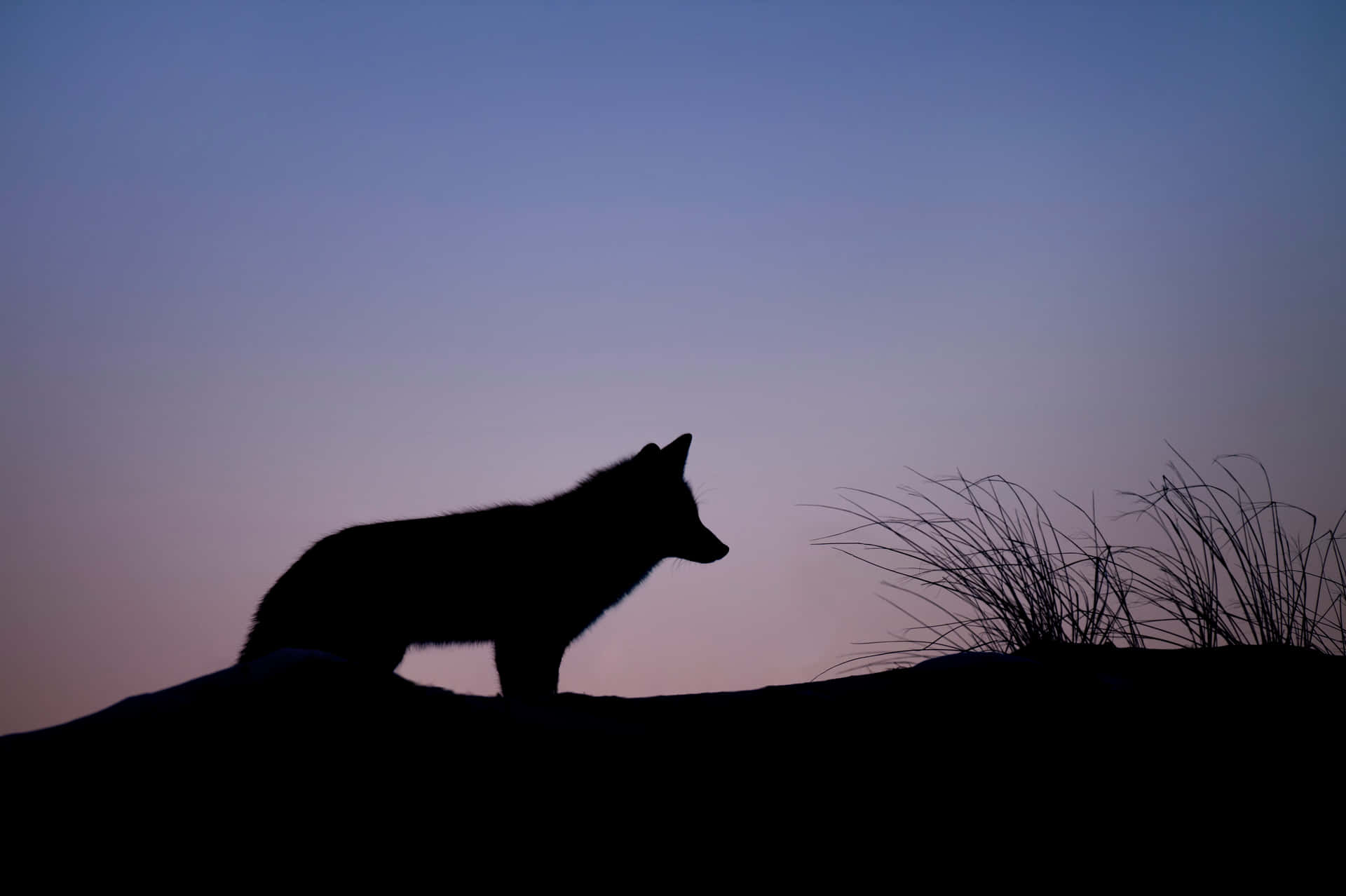In this twilight scene, the dark, silhouetted figure of a wolf stands still on uneven ground, centered towards the bottom left of the image. The wolf's profile is clearly visible with its snout pointing to the right, ears perked up, and its tail sloping downwards. Wispy tall grasses frame the silhouette to the right. The sky transitions from a bright blue at the top, blending into lighter blue hues, and finally into a pinkish color near the horizon, creating a serene gradient behind the wolf. The backdrop contributes to the dramatic yet peaceful ambiance of the scene, which is devoid of any other objects except for the grasses.